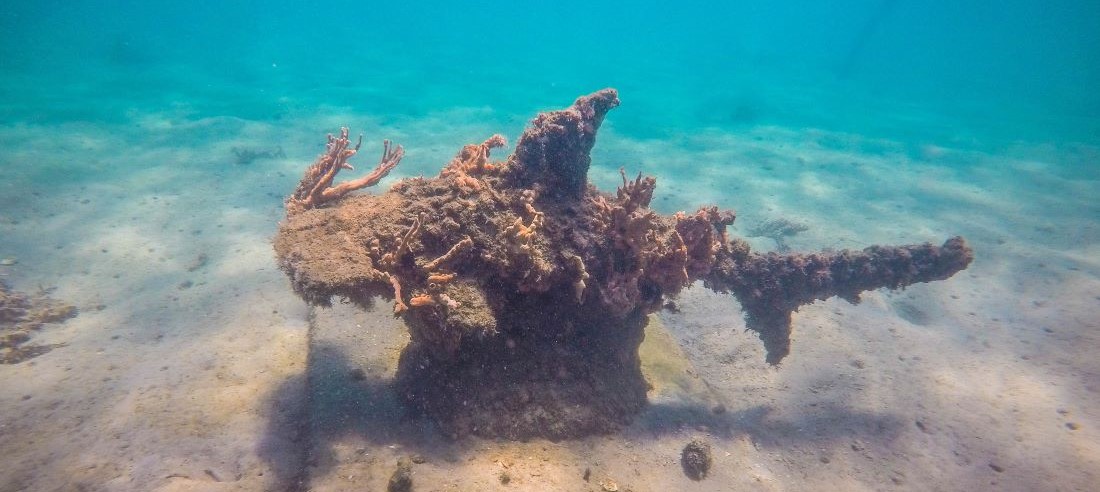Under the clear, turquoise blue waters, an intriguing structure lies on a sandy ocean floor, adorned with various sea life. This object, possibly made of metal or concrete and shaped somewhat like a hammerhead shark with a tail fin off to the right, has a bulky, thick appearance. Covered in brown and orange coral, the structure features a square base from which a rounded section arises, hinting at a prolonged submersion. Green algae, seaweed, barnacles, and small creatures with feelers and tiny eyes are attached, enriching the marine ecosystem. The light beige sand, sprinkled with hints of yellow, stretches across the ocean bed, while sunlight penetrates faintly from above, creating a captivating underwater tableau.